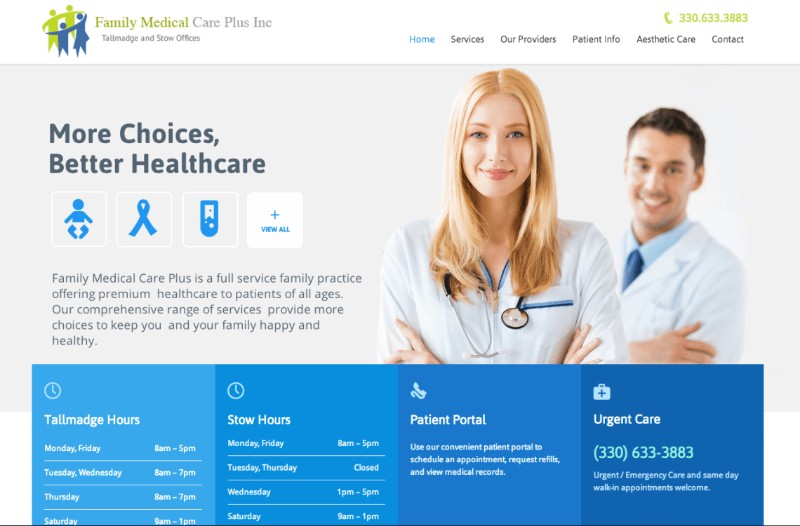The image showcases a webpage with a clean and professional design, predominantly featuring white, gray, and blue colors. In the upper left corner, the header displays the name "Family Medical & Green Care Plus, Inc." in gray text, followed by the locations "Talmadge and Stowe Offices" in smaller text below. An icon depicting two adult figures and two children, rendered in a simple, animated style, is also visible.

On the top navigation bar, there are several menu options including "Home" (which is currently highlighted in blue), "Services," "Our Providers," "Patient Info," "Aesthetic Care," and "Contact." Above these options, a contact phone number, "330-633-3883," is prominently displayed.

As you scroll down, there's a section with a gray background that reads "More Choices, Better Health Care." This section features icons representing a baby, a ribbon, and a tube, alongside a button labeled "View All" with a plus sign. The text within this section emphasizes that Family Medical Care Plus offers full-service family practice healthcare to patients of all ages, highlighting their comprehensive range of services designed to keep families happy and healthy.

To the right of this text, there is a photograph of two smiling healthcare providers: a blonde female doctor in the foreground and a male doctor with short brown hair standing behind her.

Below this, the hours of operation for both the Talmadge and Stowe offices are listed. Talmadge hours are detailed as:

- Monday through Friday: 8 a.m. to 5 p.m.
- Tuesday and Wednesday: 8 a.m. to 7 p.m.
- Thursday: 8 a.m. to 7 p.m.
- Saturday: 9 a.m. to 1 p.m.

Stowe hours are:

- Monday through Friday: 8 a.m. to 5 p.m.
- Tuesday and Thursday: Closed
- Wednesday: 1 p.m. to 5 p.m.
- Saturday: 9 a.m. to 1 p.m.

Towards the bottom of the page, there are sections for a patient portal and urgent care, both displaying the number "330-633-3883" for easy access.